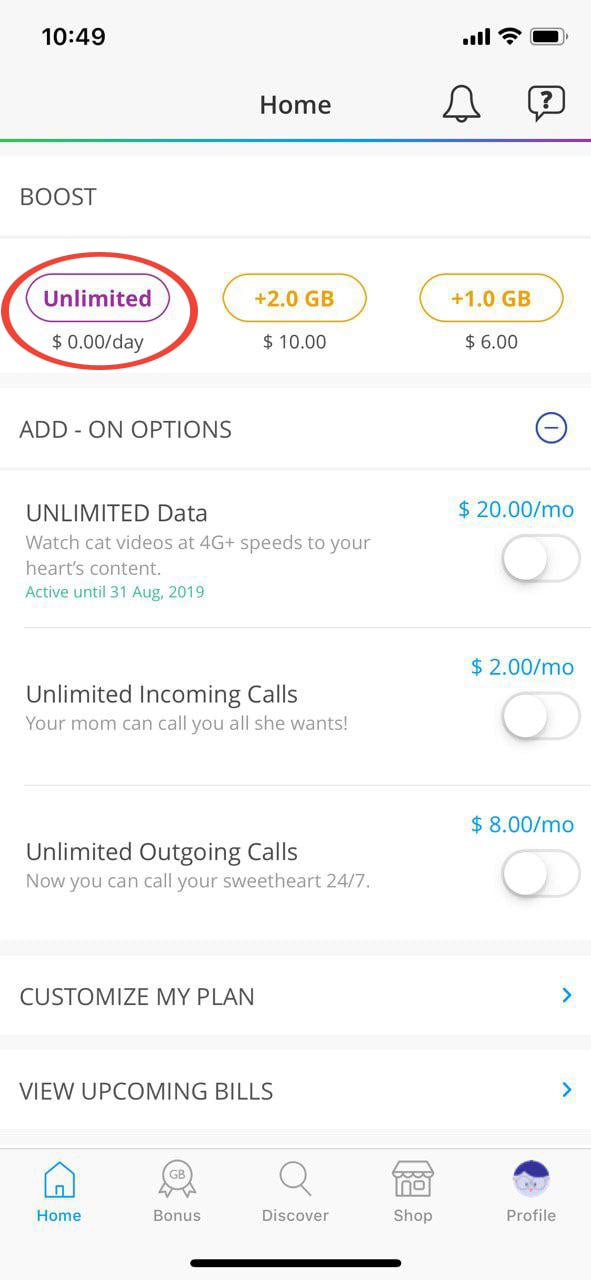This is a detailed digital screenshot of a mobile interface with an assortment of features visible on the screen. The current time is displayed as 10:49, located near indicators for the home screen, a notification bell, and a nearly full battery icon. Wi-Fi connection bars are also visible along with a question mark icon. Below these icons is the "boost" section, which offers various data plans and add-ons.

The first option available is "Unlimited" for $0 a day. To the right, there are additional data options: an extra 2.0 gigabytes for $10, and an extra 1 gigabyte for $6.

Further down, there are add-on options displayed with detailed descriptions:
- "Unlimited data" allows the user to watch CAD videos at 4G plus speeds, active until August 31st, 2019, for $20 a month. This option is not selected.
- "Unlimited incoming calls" lets your mom call you as much as she wants for $2 a month. This option is also not selected.
- "Unlimited outgoing calls" enables you to call your sweetheart 24/7 for $8 a month. This option is unchecked as well.

Finally, there is an option to "Customize my plan," allowing further tailoring of the mobile service plan.